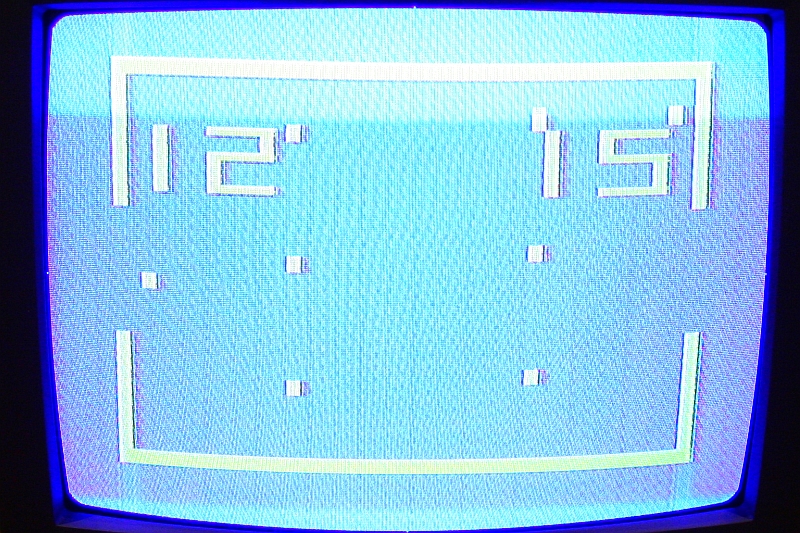The image features an old CRT television displaying a game of Pong. The photograph itself, rather than a direct screenshot, reveals the characteristic horizontal lines often seen when capturing images of CRT screens. The game is actively in progress with the left player's score at 12 and the right player's score at 15. The screen's background is predominantly light blue in the center, transitioning to dark blue around the edges, with the Pong game elements rendered in white. The television's frame is black, and only the screen is visible, with no other features of the TV shown in the image.